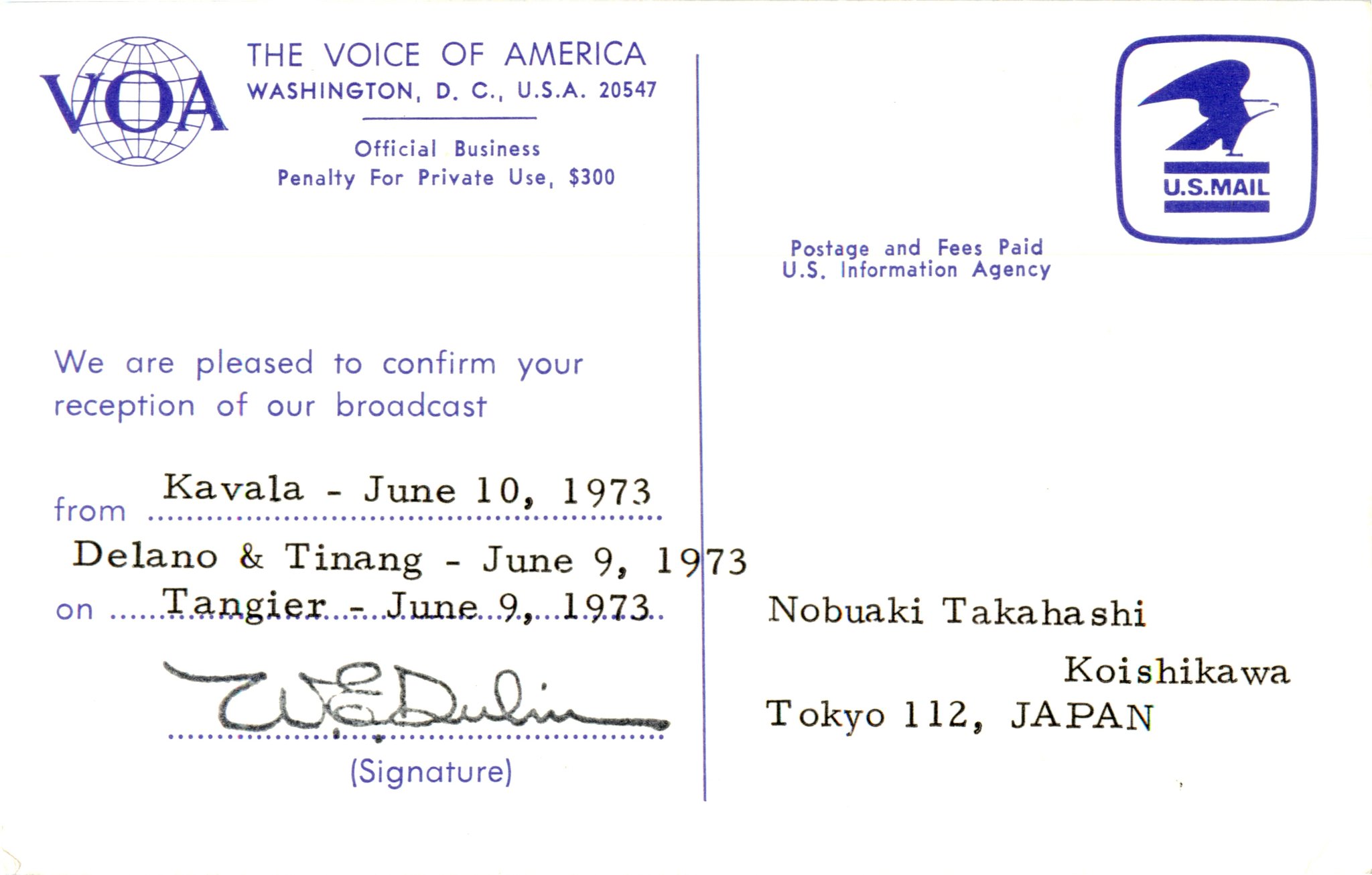This image displays the back of a postcard divided by a thin vertical blue line. The left side features multiple text elements: at the top left is a globe icon with "VOA" inscribed on it, followed by the text "The Voice of America, Washington, DC, USA 20547." Below this, it reads "Official business, penalty for private use $300." Further down, the postcard confirms the reception of broadcasts from Kavala on June 10, 1973, Delano and Tinang on June 9, 1973, and Tangier on June 9, 1973, each filled in by typewriter. Beneath this, there's a handwritten signature. The right side of the postcard exhibits a U.S. Mail logo with a blue border in the top right corner. To the left of the logo, it states "Postage and fees paid, U.S. Information Agency." Below this, the recipient's details are typed: "Nobuaki Takahashi, Koishikawa, Tokyo 112, Japan." The background of the postcard is white.